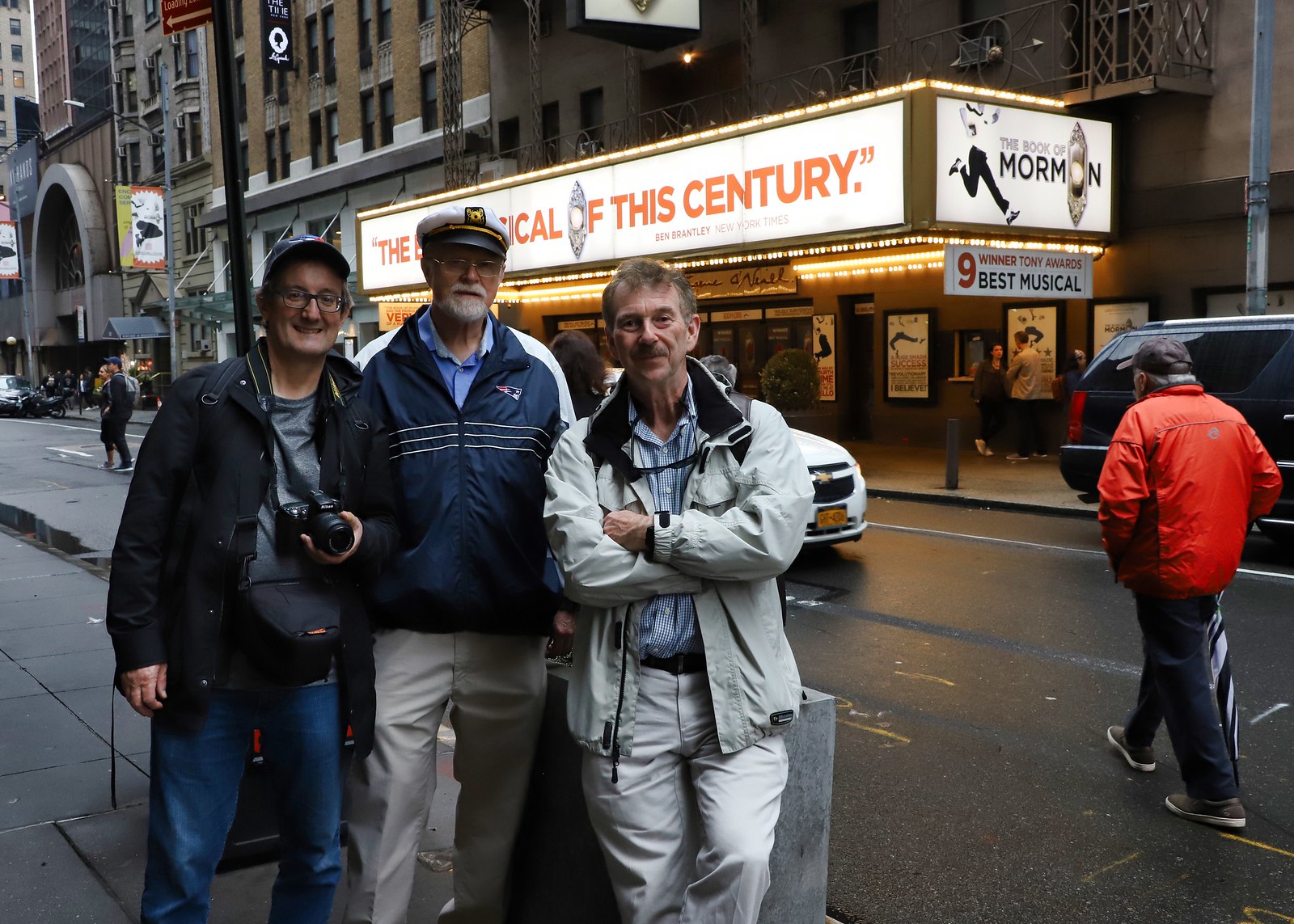In an outdoor daytime photograph, three older men stand together in front of a theater, posing for a picture on an asphalt street. The man on the left wears a black baseball cap, glasses, a dark blue jacket, a gray shirt, and blue jeans. He smiles as he holds a camera that hangs from a strap around his neck. The man in the middle sports glasses and a white sea captain's hat, with a gray mustache and goatee. He wears a blue New England Patriots sweatshirt under a blue zip-up windbreaker and light khaki pants. The man on the right, with light brown hair and a mustache, stands with his arms crossed over his chest, wearing a light gray jacket over a blue and white checkered shirt and khaki pants. A man in a red jacket walks past them on the right side of the image.

Behind the men, a large billboard with a white background partially obscures its text, but it prominently displays "The Musical of This Century" and highlights "The Book of Mormon" along with a banner recognizing "Winner of 9 Tony Awards, Best Musical." The street behind them is lined with various vehicles, including a white car directly behind the group and a dark SUV parked further down the road. A gray streetlight pole also stands nearby, adding to the urban backdrop.